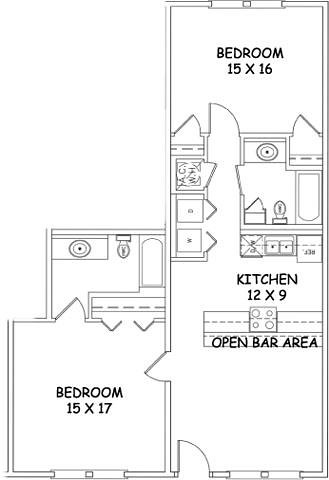This detailed computer-designed sketch showcases the layout of a multi-room apartment. The primary structure is a large rectangle, divided into distinct living spaces. On the right side, there is a long, narrow rectangle. Adjacent to the bottom of the main rectangle on the left, there's a smaller square which is parallel to it. Above this smaller square is an additional rectangle indicating a second bathroom.

Starting at the top of the large rectangle, labeled as "Bedroom," the space measures 15x16 feet. Directly below, there's a bathroom fully equipped with a bathtub, toilet, sink, shower, and spaces allocated for a washer and dryer, along with an AC unit.

This seamlessly transitions into the kitchen area, which is 12x9 feet, containing a refrigerator, sink, and stove positioned opposite to each other. An open bar area connects to the bottom part of the main structure.

On the left-hand side, a smaller square indicates another bedroom, measuring 15x17 feet. A door from this bedroom opens into an adjacent tiny bathroom, compactly designed with a bathtub in the top right corner, followed by a toilet and a sink.

The sketch meticulously delineates the apartment's spatial arrangement and amenities, providing a clear and comprehensive overview of the interior design.